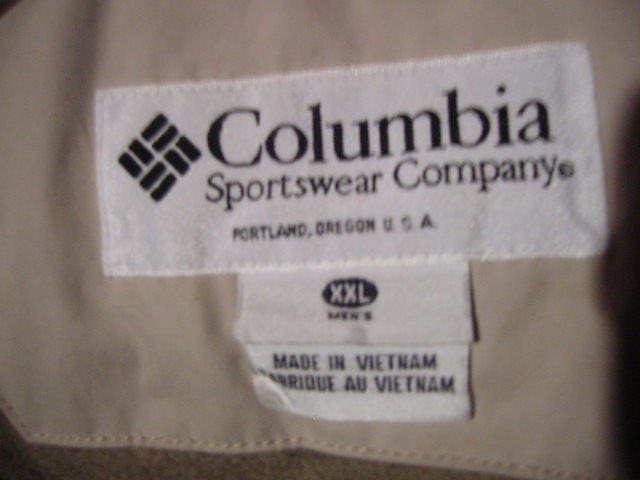This detailed caption describes the labels inside a Columbia Sportswear Company waterproof jacket:

"The image features the interior tags of a waterproof jacket from Columbia Sportswear Company. Centrally sewn onto the beige lining of the jacket is a white fabric tag, affixed flatly against the back portion of the jacket. The tag prominently displays the Columbia Sportswear Company logo, accompanied by the trademark symbol (™) encircled to the left. Below the 'Columbia' name, the words 'Sportswear Company' are clearly printed.

Adjacent to this main tag, there is a separate hanging tag indicating the size 'Xtra Xtra Large' or 'XXL.' Another hanging tag beneath it states 'Made in Vietnam,' followed by the phrase 'Fabriqué au Vietnam' in another language, showcasing the country of origin. The brand's recognizable trademark diamond shape, which includes a pattern of different square-like images, is also visible on the sewn tag. The jacket's outer material appears beige and is complemented by a lining underneath, reinforcing the waterproof quality of the garment."